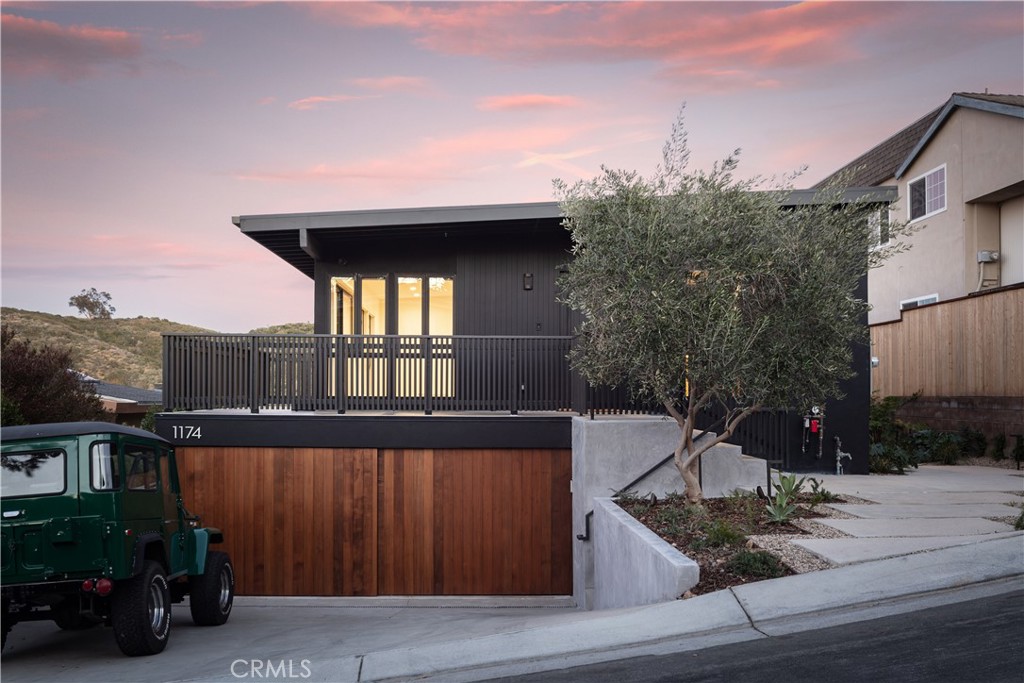The image captures a serene residential scene taken at either sunrise or sunset, evident from the sky's soft pink hues. The foreground features a black-and-gray house with a distinct wooden garage door made of bright brown slats. The house boasts a gray railing and four vertical windows, framed centrally in the photo. In the driveway, a green Jeep with the registration number '1174' is parked. An olive tree is positioned near the garage, complementing the stone pathway that leads up to the house. The surrounding neighborhood and hills can be seen in the backdrop, with a beige house neighboring the main residence. The image, watermarked CRMLS, provides a horizontal landscape orientation of this tranquil setting.